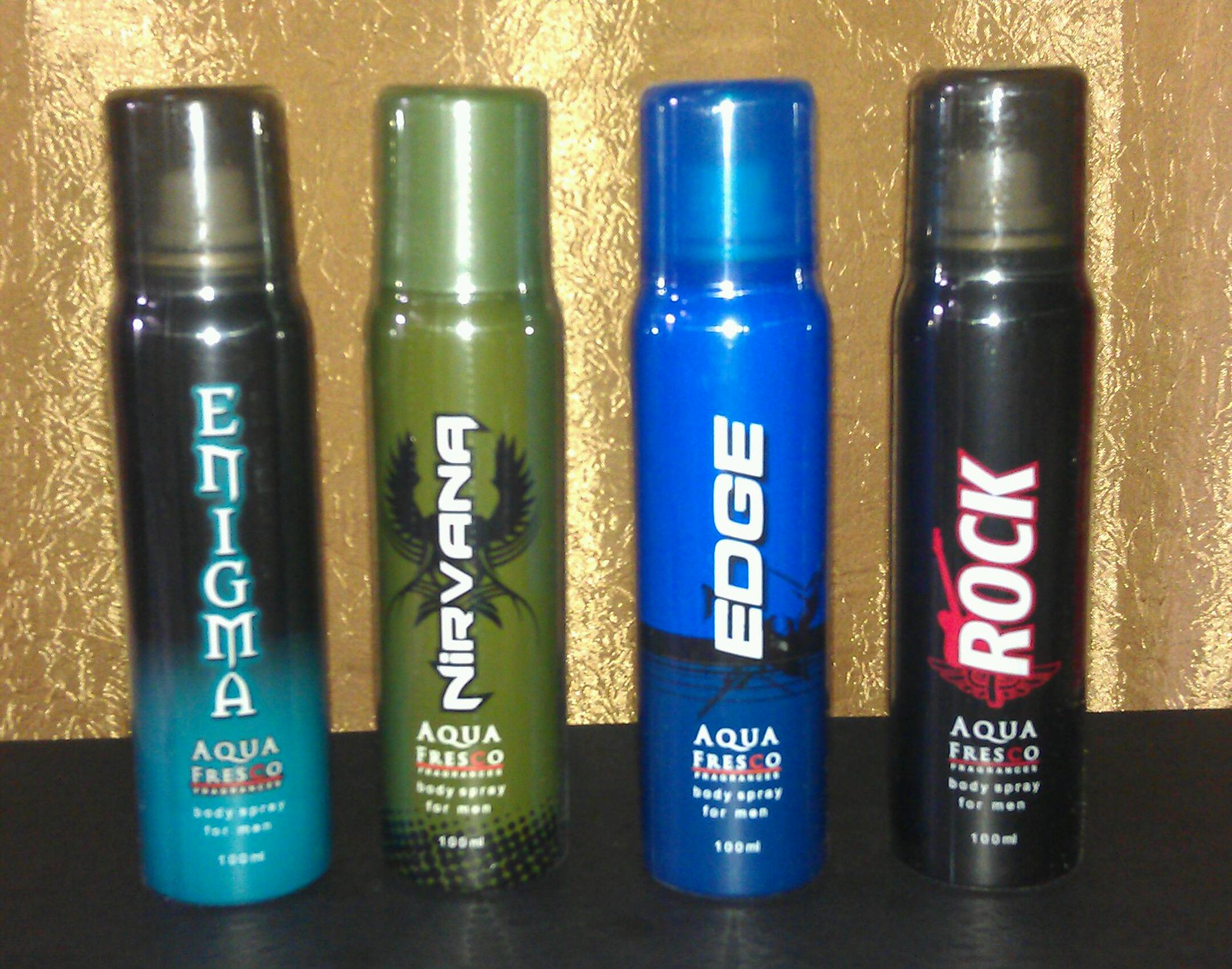This color photograph displays four distinct cans of Aqua Fresco body spray for men, neatly arranged on a black tabletop with a shiny gold foil backdrop. From left to right, the first can is black fading into turquoise and prominently features the word "Enigma" in a vertical blue and white font. It advertises Aqua Fresh body spray for men. The second can, a camo green color, is labeled "Nirvana" with white letters ascending from the bottom, accompanied by an image of an eagle. It also lists Aqua Fresco Body Spray for men. Next, the bright blue can displays the name "Edge" in white lettering running upwards and similarly states Aqua Fresco body spray for men. The final can, predominantly black, highlights the word "Rock" in ascending order with a red guitar graphic in the background, completing the lineup of Aqua Fresco body sprays for men, each holding 100 milliliters.